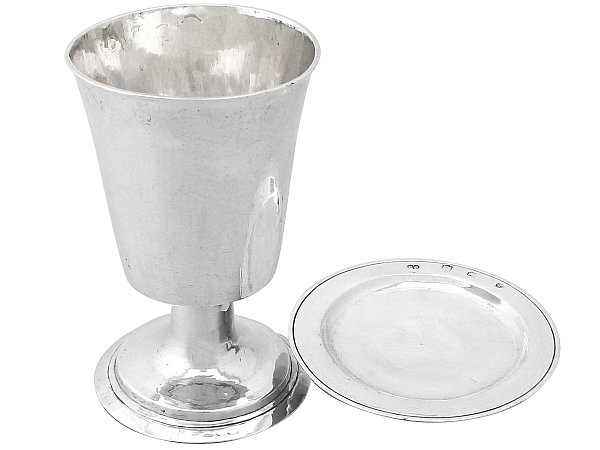The image depicts a highly reflective, silver goblet with a chrome finish, standing on a flat, somewhat conical base adorned with a few ridges. The goblet narrows as it extends down to the base and features a thicker stem. Next to the goblet is a silver plate, just wide enough to accommodate the base of the goblet. This plate has a black circular line near its edge and some indiscernible black spots on the right-hand side, accompanied by white highlights and subtle shadows. The underside of the goblet’s base displays a series of small symbols: the first resembles a spout of water, the second an upward arc, the third possibly a sea motif, and the fourth is circular with a rough texture. The entire setup is displayed against an all-white background, emphasizing the goblet's shiny chrome finish both inside and out.